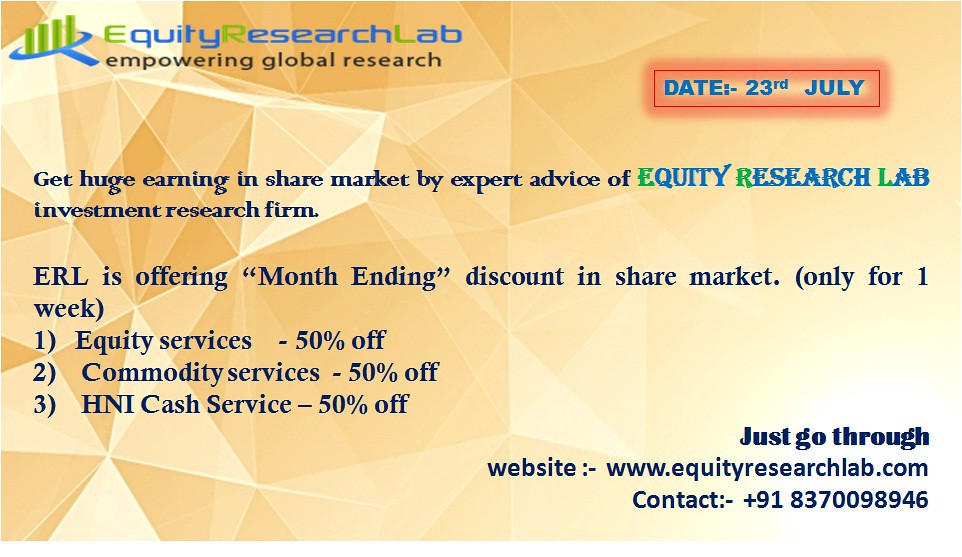The image depicts a promotional advertisement for the Equity Research Lab, an investment research firm, set against a tan, multi-colored background featuring shades of orange, green, blue, pink, yellow, and white. The composition is done in landscape mode, filling the entire image area. 

In the top left corner, the firm's logo is presented with four vertical green rectangles leading to a blue circle, alongside the text "Equity Research Lab" with "E," "R," and "L" in green and the remaining letters in blue. Below the logo, the company’s tagline "Empowering Global Research" appears in black.

A red outlined rectangle in the upper right corner, though slightly blurred, contains the date "23rd July." Adjacent to this, a headline reads "Get Huge Earnings in Share Market by Expert Advice of Equity Research Lab, Investment Research Firm," with the same green and blue color scheme for "Equity Research Lab."

Further down, a promotional message in navy blue or black text announces, "ERL is Offering Month-Ending Discount in Share Market Only for One Week." This is followed by a list:
1. Equity Services - 50% Off
2. Commodity Services - 50% Off
3. HNI Cash Service - 50% Off

In the lower right-hand corner, highlighted in white, there is a call-to-action urging users to "Just go through" with subsequent details including the website "www.equityresearchlab.com" and the contact number "+91-837-009-8946," both printed in blue.

The advertisement aims to drive traffic to their website and promote limited-time discounts on various financial services, using a visually engaging and colorful design.